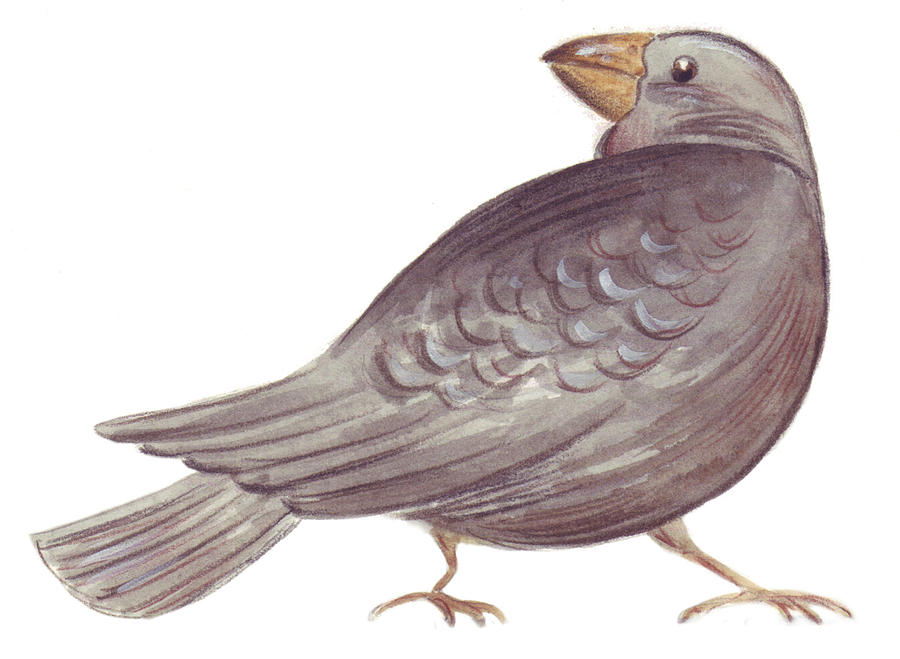This artwork is a detailed, colorful drawing of a bird, possibly a robin or mockingbird, characterized by its rounded body and vibrant mix of hues. The bird is mostly rendered in shades of gray, from dark charcoal to bluish-gray, with some lighter tints suggesting a potential use of colored pencils or pastel colors. Its body is oriented to the right, but its head is intriguingly turned 180 degrees to face left, giving the bird a watchful appearance. The bird's legs are depicted in a tannish-brown, firmly planted on the ground, adding to its lifelike stance despite the simple, somewhat stylized nature of the drawing. The beak is a notable feature, painted in a yellowish-orange hue, contrasting with the black eye which adds a touch of realism. The entire bird is set against a plain white background, offering no additional context beyond its own vivid portrayal.